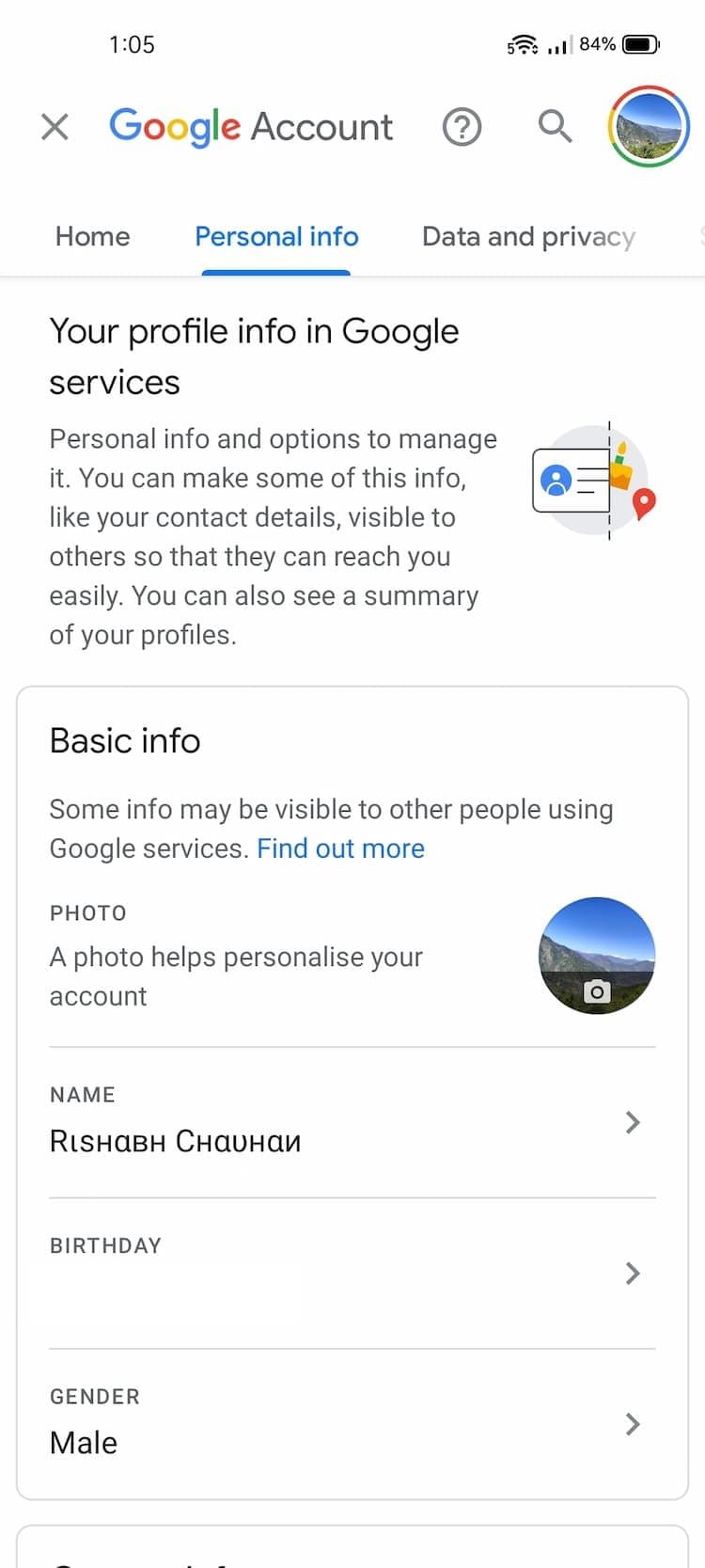The image depicts a mobile app landing page with various UI elements and personal information management options. 

At the top left corner, the time is displayed as 1:05. In the top right corner, there are icons showing full Wi-Fi signal, three out of four bars of cellular signal, and an 84% battery life indicator.

Below this status bar, from left to right, are an 'X' icon, a Google account icon, a question mark, a magnifying glass, and the user's avatar. The Google logo appears in its characteristic blue, red, yellow, blue, green, and red color scheme.

Underneath the Google logo, three menu options are visible: "Home," "Personal info," and "Data privacy." The "Personal info" option is currently active, indicated by blue text and an underline.

The main section starts with the heading, "Your profile info in Google services," followed by smaller text explaining that personal information and options to manage it are available. It states that some contact details can be made visible to others for easier communication, and users can also view a summary of their profiles. To the right of this text, there is an illustration resembling an identification card, featuring a birthday icon, a red pin indicating address or location services, all contained within a circle.

Below this section is a rounded rectangular box with various options. The box's header reads "Basic info" in large text, and underneath is smaller text that says, "Some info may be visible for other people using Google services. Find out more," with "Find out more" as a hyperlink. 

Additional options within this box include:
- "Photo," with a prompt to personalize the account, alongside the user’s avatar, which is a mountainscape with a larger mountain on the left side.
- "Name," displayed in what seems to be Russian or another Eastern European language.
- "Birthday," currently left blank.
- "Gender," listed as male.

Each of these options has a right arrow on the right side, indicating that they are editable fields.